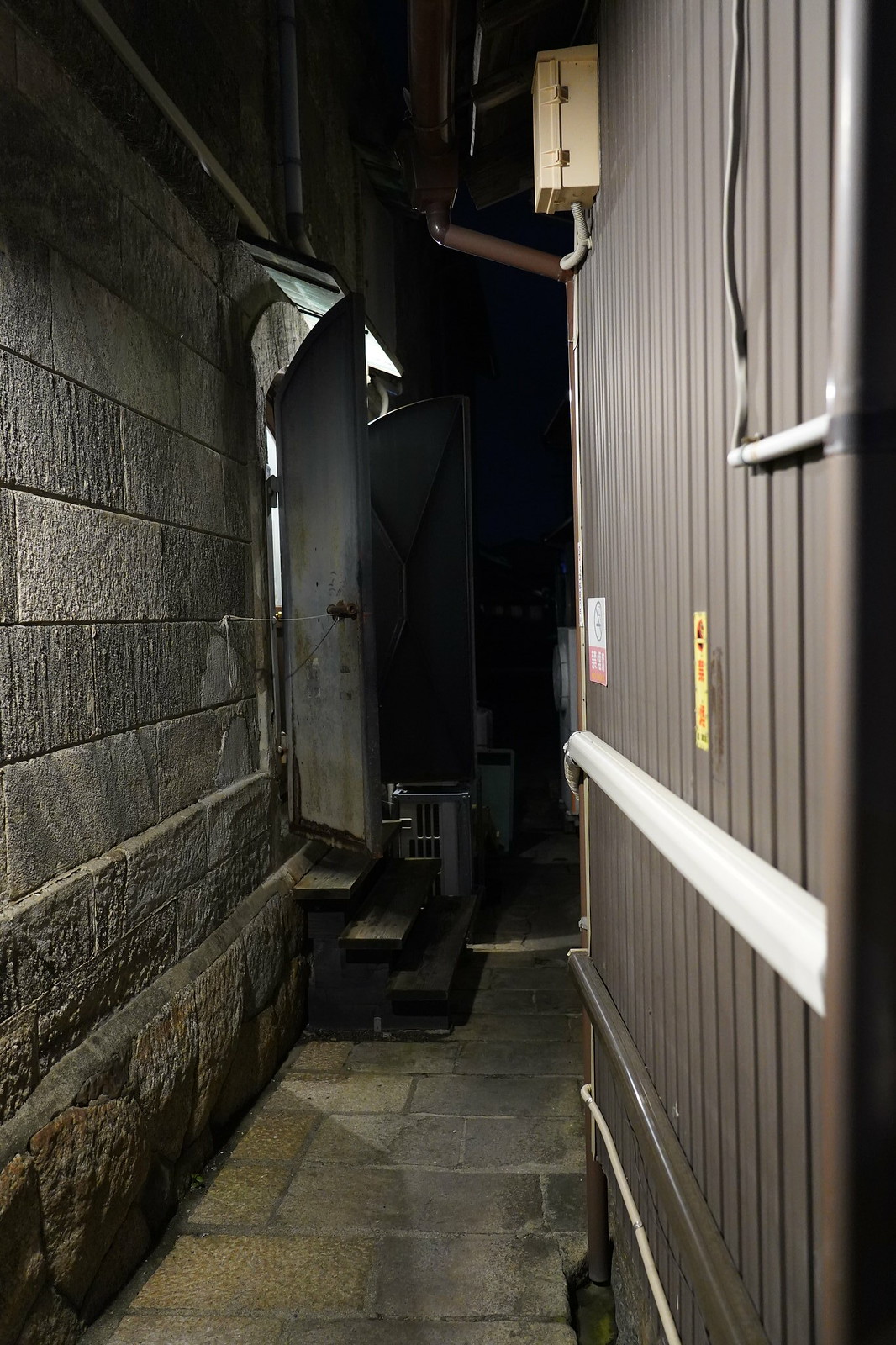The image depicts a narrow alleyway at nighttime, illuminated by an unseen light source, which brightens the scene while leaving the background dark. The ground is covered with cemented stone bricks that run through the center of the image. On the left side, there is a gray brick or cinder block wall featuring a small staircase of three steps leading up to a slightly open metal door, possibly indicating an entry to a business or company. An air conditioner unit is situated next to this door. To the right, a brown wooden panel structure with vertical lines and a white piece of wood across it can be seen, possibly functioning as a wall or fence, with pipes running along its surface, including a brown vertical pipe. Despite the mix of shades—gray, brown, yellow, red, orange, and tan—the image remains clearly devoid of any textual elements.